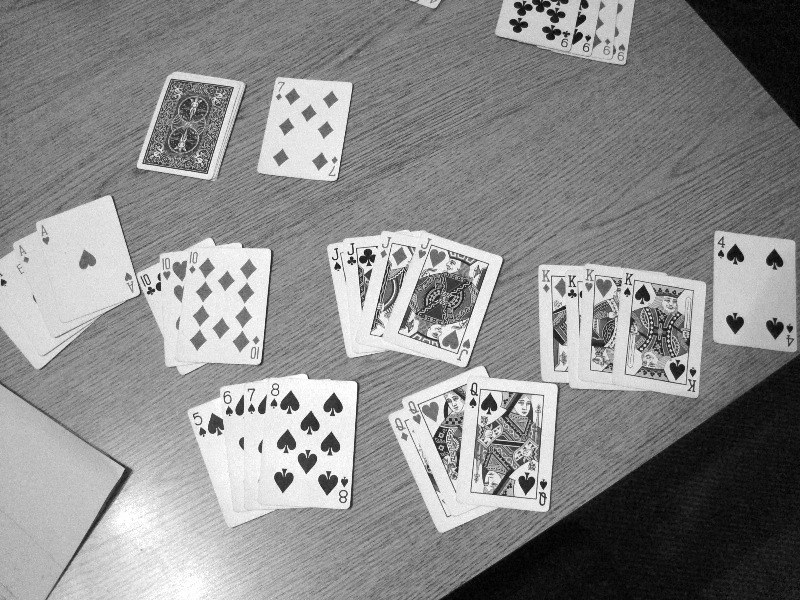A meticulously arranged scene on a polished, lightly finished plywood table, captured in black and white. Atop the table lie several neatly organized piles of standard playing cards. Each pile is sorted by ranks: four kings, four jacks, three queens, three tens, and four aces. Another pile sequentially orders the numbers five through eight, while a solitary four rests in a corner. The table is slightly cropped in the photo, suggesting the photographer's perspective from above. On one side, a paper folder or notes are barely visible, and on the opposite edge, the corner of another pile of cards hints at a second participant, possibly engaged in an intricate card game.